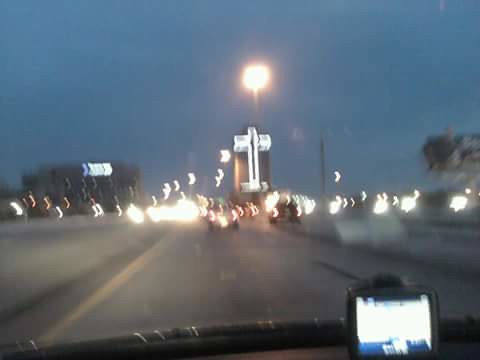Photograph taken from inside a vehicle through the windshield shows the partial black dashboard at the bottom, featuring a mounted phone or GPS holder. In the distance, numerous cars can be seen driving away, their lights creating a trail. On the left side of the road, a gray cinder block barrier runs parallel to a solid yellow line. Dominating the center of the image is a large, illuminated white cross affixed to a multi-story building. Above it, against a backdrop of blue sky, is what appears to be either a street light or the moon. On the far right, trees are visible, and the overall scene has a blurry quality, causing the lights ahead to bend towards the left. Another multi-story building is also visible on the left side of the image.